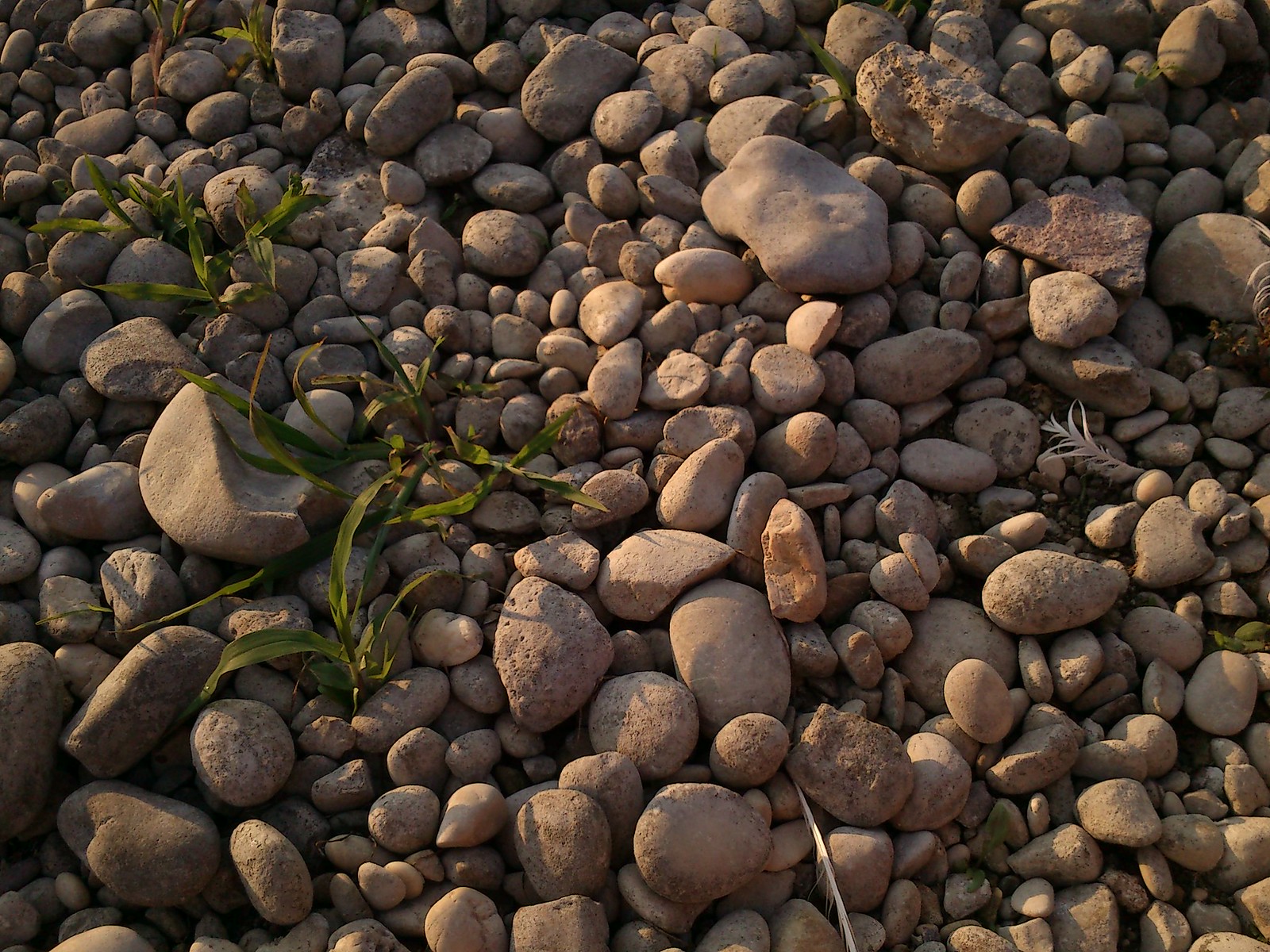The image showcases a dense collection of stones of various shapes, colors, and sizes. Predominantly occupying the entire frame, these stones range from small pebbles to larger rocks that overlap each other. The stones exhibit a diverse palette including shades of tan, brown, white, black, copper, light gray, dark gray, reddish, and bluish hues. Among the mostly smooth and round stones, there are also oblong, half-circle, and non-specific shaped rocks. Sparse green weeds and grasses can be seen sprouting through the gaps between the stones, primarily on the left side of the image, with some sticks interspersed as well. The scene appears to be outdoors on a rocky beach, captured in daylight. There is no visible text in the picture.